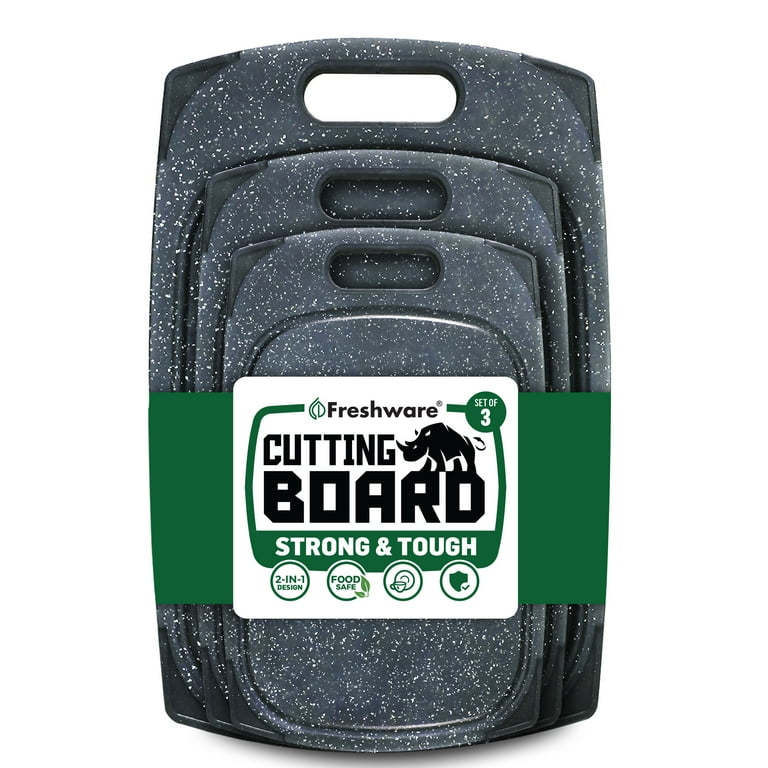This image showcases a set of three cutting boards of varying sizes, artfully nested together and packaged with a dark green cardboard label at the bottom. The cutting boards are predominantly black with a unique lighter black shade and white polka dot design. The smallest board is on top, followed by the medium-sized one, and the largest at the bottom, with the top cutting board featuring dark black upper corners. Each board is equipped with a handle and groove marks for efficient use. The packaging includes a prominent white label with green edges, proclaiming "Cutting Board Strong and Tough" and features the brand name "Freshware" along with a rhinoceros logo. Below the slogan, there are four icons: a two-in-one design, a food-safe indication with green leaves, a cup and saucer graphic, and a shield with a check mark, all set against a plain white background.